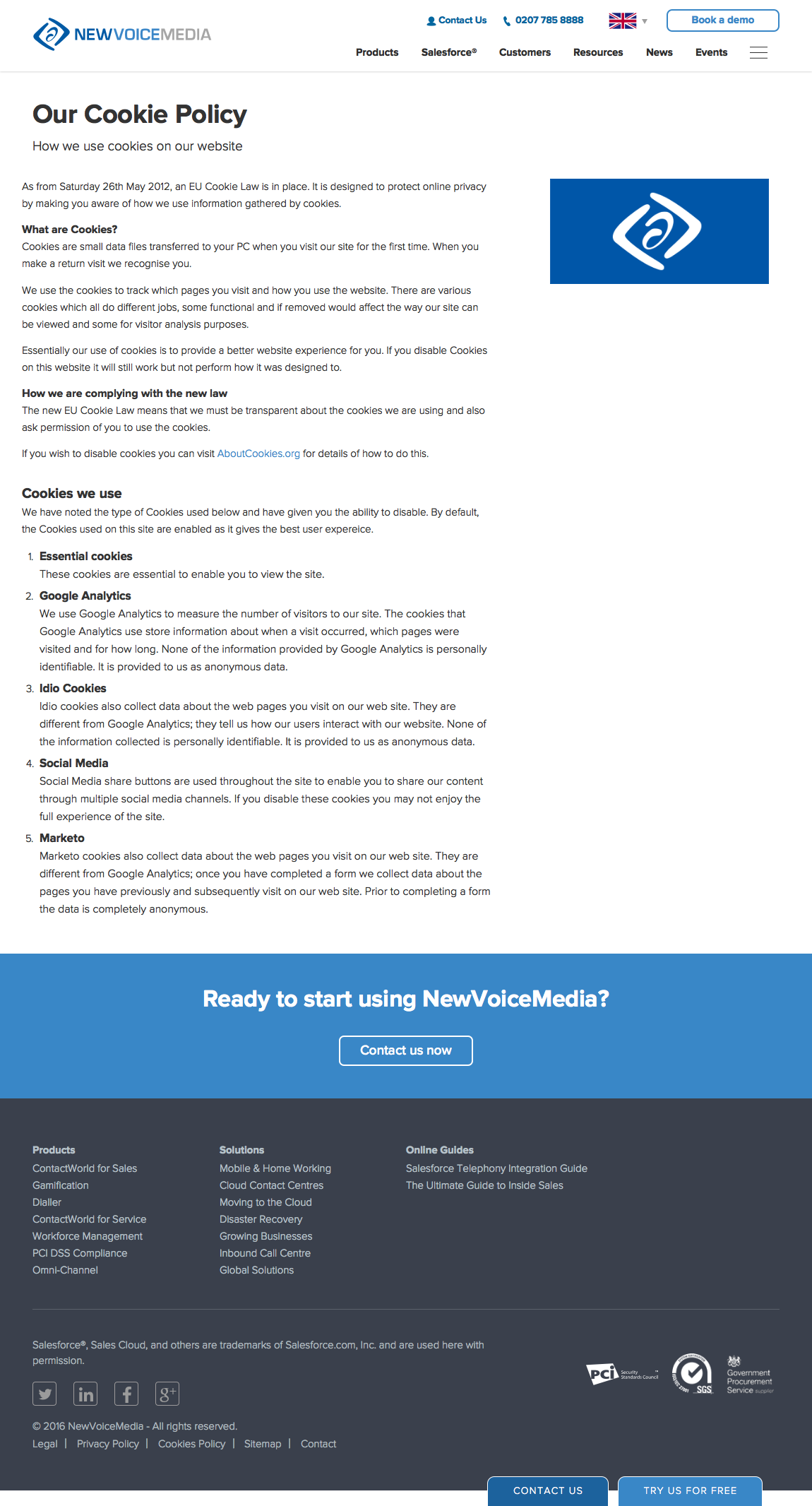Screenshot of a New Voice Media Web Page

This screenshot captures the top section of New Voice Media's website and features a meticulously organized navigation menu. At the very top, there are several options: Products, Salesforce, Customers, Resources, News, and Events. On the extreme top-right is a "Contact Us" option alongside a phone number, 0207-785-8888, and a United Kingdom flag indicating the regional setting. Adjacent is a prominent "Book a Demo" button.

The webpage also outlines details of the cookie policy, specifying types such as essential cookies, Google Analytics, video cookies, and social media cookies. On the right side, the New Voice Media logo is prominently displayed within a blue box.

Beneath the cookies description is a blue banner encouraging users to start using New Voice Media with a "Contact us now" call to action. Scrolling down, a black banner presents what seems like a site map. The left section lists various products including Contact World for Sales, Gamification, Dialer, Contact World for Service, Workforce Management, PCI DSS Compliance, and Omni Channel.

The central column focuses on solutions, highlighting Mobile and Home Working, Cloud Contact Centers, Moving to the Cloud, Disaster Recovery, Growing Businesses, Inbound Call Centers, and Global Solutions.

To the right, there's a collection of online guides including the Salesforce Telephony Integration Guide and The Ultimate Guide to Inside Sales. Beneath these guides, there are legal statements about Salesforce trademarks and social media icons for Twitter, LinkedIn, Facebook, and Google Plus.

At the webpage's footer, there’s a copyright notice from 2016 stating "New Voice Media, all rights reserved." Alongside, it offers options for Legal, Privacy Policy, Cookies Policy, Site Map, and Contact. Finally, at the very bottom-right corner, there are two blue buttons: "Contact Us" and "Try Us for Free," accompanied by additional legal icons.